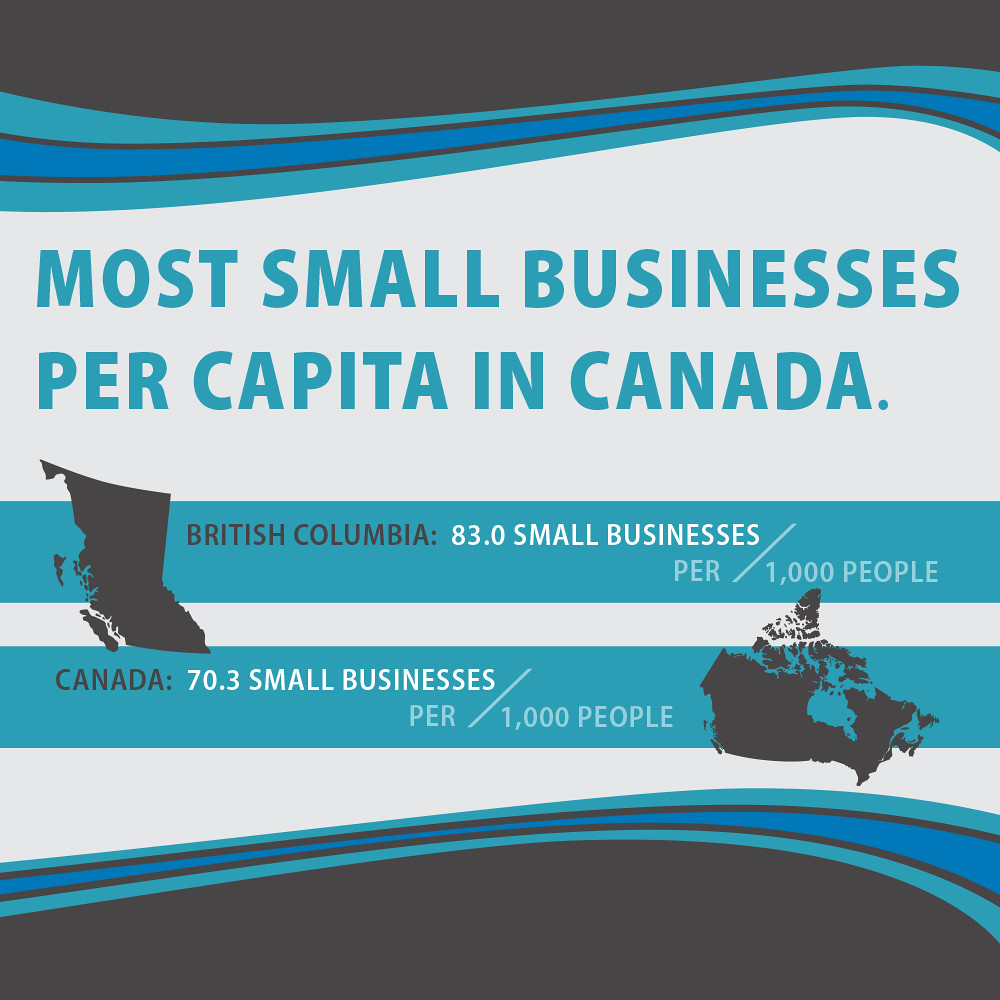The promotional flyer, designed in a square format with a color palette of white, blue, aqua, and black, highlights statistics about small businesses in Canada. At the top, a curvy black banner is followed by an aqua swirl and a blue swirl. Below this decorative header, bold text in blue font announces: "MOST SMALL BUSINESSES PER CAPITA IN CANADA." Centered beneath this header, a blue horizontal stripe showcases an image of British Columbia on the left, reading: "British Columbia: 83.0 small businesses per 1,000 people" in black and blue fonts. Below this, a slimmer white stripe and a larger blue horizontal stripe display the national statistic: "Canada: 70.3 small businesses per 1,000 people," accompanied by a black silhouette of Canada. The flyer concludes with a mirrored decorative band of aqua and blue swirls at the bottom, contributing to its cohesive graphic design.